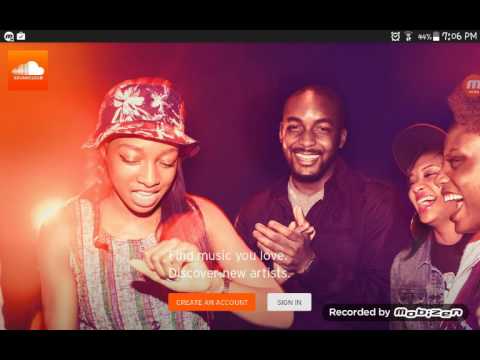This image captures a moment on a music streaming site, likely SoundCloud, given the presence of its logo—a white cloud on an orange background—in the upper left-hand corner. The time displayed at the top is 7:06 p.m., with battery life at 44% and an alarm clock icon next to it. The image quality is low, showing significant pixelation and compression artifacts. 

At the bottom of the screen, there is text reading "Recorded by Mobizen," with the letters M-O-B-I-Z-E-N in an alternating raised and lowered pattern, overlaid on a semi-transparent, 50% screened capsule shape. 

In the center of the image, there is a photograph featuring four African-American individuals. The person on the far left is a girl wearing a flower-printed bucket hat and a sleeveless top that appears to be either plaid or striped. She has her left hand bent and raised in front of her chest, possibly indicating that she is singing or engaged in conversation. 

Next to her, a man dressed in a black shirt over a white undershirt appears to be clapping. To his right, two women are visibly enjoying the moment, both facing left and seemingly laughing hysterically. The more visible woman is wearing a baseball cap and a jean jacket. The woman on the far right has voluminous curly hair, but her outfit is largely obscured. The overall scene suggests a lively, spontaneous moment, perhaps during a music recording or playback session.